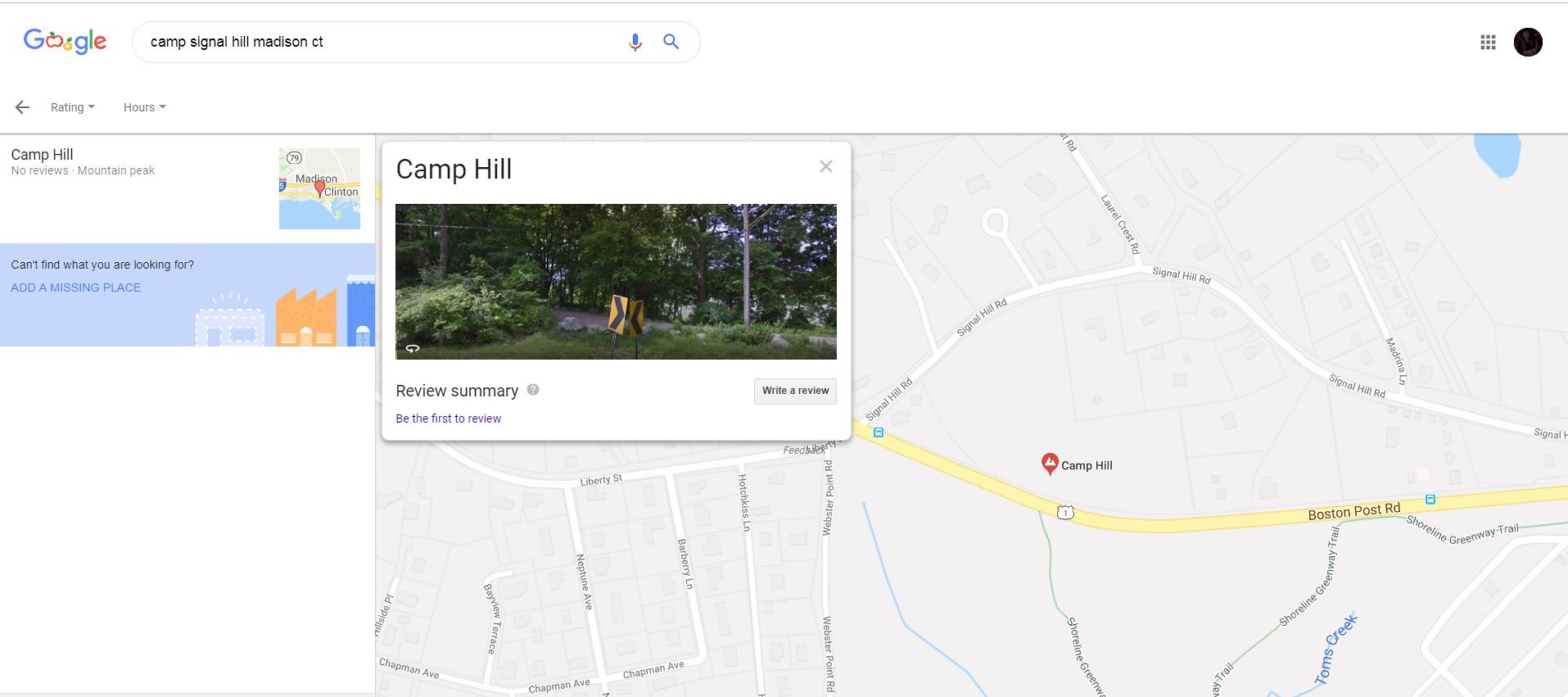This screenshot captures a detailed Google search result for "Camp Signal Hill Madison CT."  Positioned at the top left is the Google logo, with the distinctive blue, red, and yellow letters. However, in this instance, the O’s are creatively replaced with a larger red apple and a smaller yellow apple. To the right, the search bar displays the queried text, while across from it on the top right, there are navigation icons including a grid of nine dots for a menu and a dark circle placeholder for a profile picture.

The page is in light mode, featuring a white background. Directly below the search bar, the left toolbar includes options marked "Reading" and "Hours," each accompanied by a down arrow. Dominating the middle two-thirds of the screenshot is a map pinpointing Camp Hill. The map, primarily showcasing a gray background with a yellow-highlighted road labeled Boston Post Road, features a red pin with a mountain icon marking the camp's location.

Embedded within the map is a pop-up box with an image depicting green trees, a bush, a road, and a yellow traffic sign with arrows pointing in both directions. Accompanying the map is a rectangular photograph of the campground. On the left sidebar, there is additional information about Camp Hill, including the notice "no reviews" and "Mountain Peak." Beneath that lies a small map snippet with a corresponding red pin. The sidebar extends to feature a blue call-out box stating "Can't find what you're looking for?" and includes an illustration of three cartoony buildings.